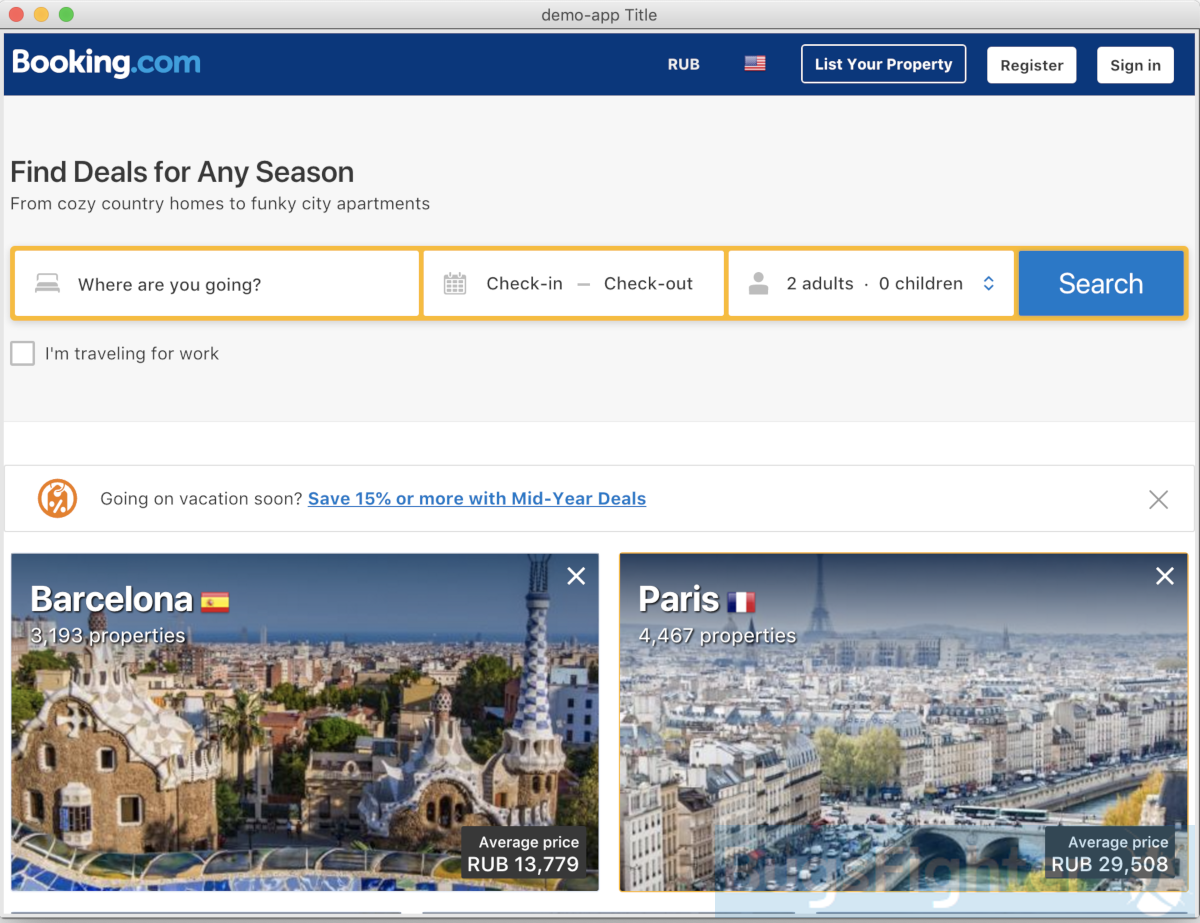This screenshot from Booking.com, captured on a Mac computer, features the distinct red, yellow, and green dots located in the upper left corner, a signature of the Mac operating system. The browser tab is titled "demo-app title." The top of the page showcases a blue banner with the Booking.com logo, indicating the currency set to Russian Ruble (RUB) and the language displayed through an American flag, suggesting US English.

Prominent buttons include a blue "List your property" button, followed by white "Register" and "Sign in" buttons. Below this, a gray block contains a banner with the message, "Find deals for any season from cozy country homes to funky city apartments," displayed in black font.

The search interface consists of several input fields and dropdown menus: "Where are you going?" and "Check-in, Check-out" with a small calendar icon, followed by options to select the number of adults and children. A blue "Search" button is also present for initiating a search. 

A checkbox labeled "I'm traveling for work" appears beneath the search section. Further down, there's a promotional banner announcing mid-year deals, offering savings of 15% or more for vacation-goers. Two destinations are highlighted: Barcelona, featuring 3,193 properties with an average price of 13,779 rubles, and Paris, offering 4,467 properties with an average price of 29,508 rubles.